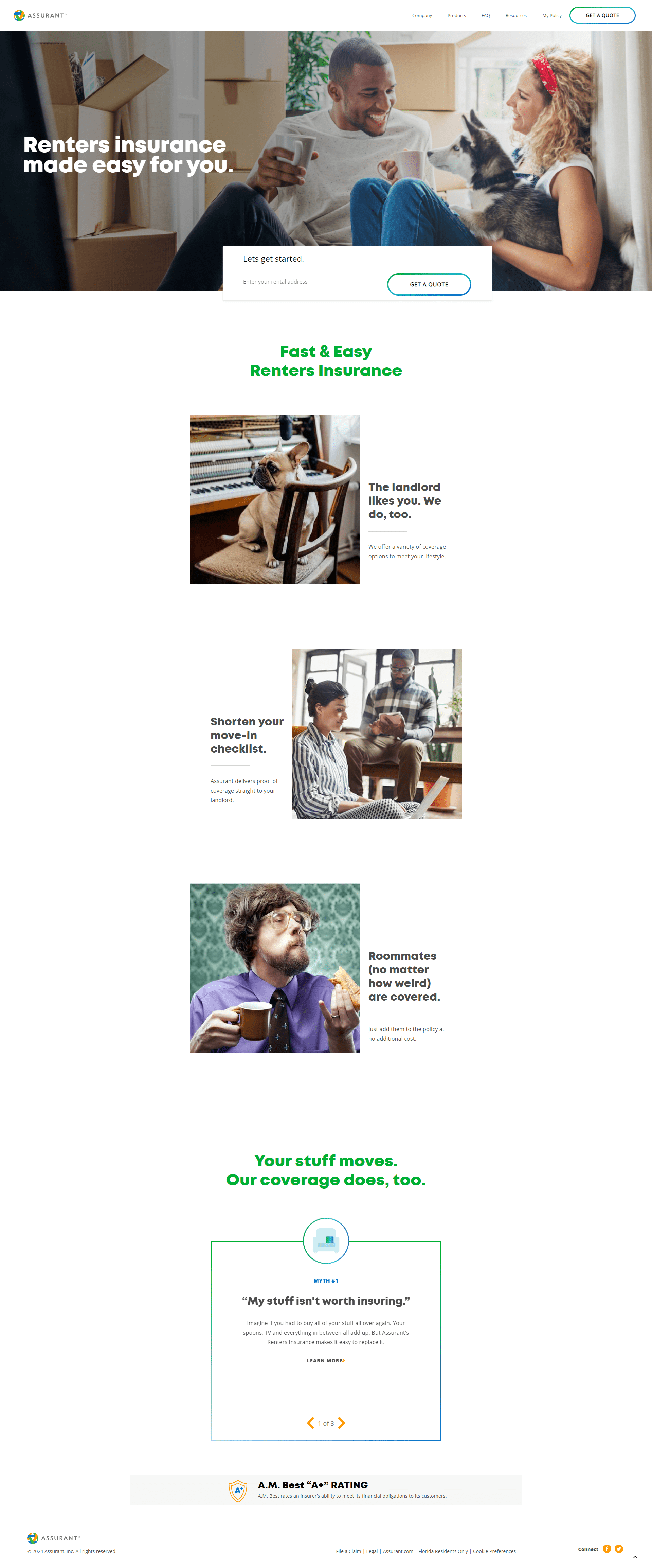Screenshot of a "Renters Insurance Made Easy" webpage:

This detailed webpage features a visually engaging background image of a cheerful couple at home, implying a sense of warmth and security that renters insurance can provide. Against the backdrop, a smiling Black man with a white long-sleeved shirt sits on the floor, holding a drink. Beside him, a blonde Caucasian woman in a red headband, jeans, and a white tank top cuddles a playful black husky puppy. Both individuals radiate happiness and comfort, seated amidst scattered moving boxes, which subtly suggests their recent move into a new rented space.

Above the image, the webpage headline reads "Fast and Easy Renters Insurance" in bold green text, appealing to potential customers looking for a smooth and quick insurance setup. Below this headline is a section with three smaller images, each depicting various home and pet scenarios: 

1. A dog sitting on a chair by a piano, complemented by a caption that mentions something about landlord approval.
2. A white woman and a Black man, both with dark hair, sitting in a room as part of a segment promoting a streamlined move-in checklist.
3. A bearded man with a quirky hairstyle, glasses, a purple shirt, and a black tie holding a cup and some food, associated with a feature about your belongings being consistently protected ("your stuff moves or covers does too").

At the very bottom of the screenshot, a blue or green-circled box pops up with the highlighted statement "My stuff isn't worth breaking," though the rest of the text within this box is obscured.

Overall, the webpage aims to convey a user-friendly and reassuring approach to renters insurance, encapsulating themes of ease, happiness, and security as it appeals to prospective customers.